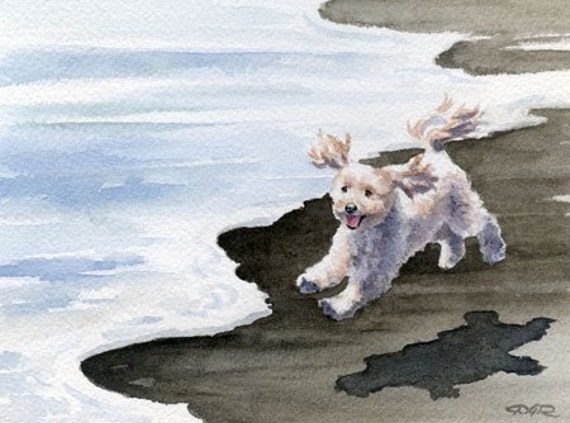This detailed watercolor painting captures a joyful beach scene featuring a small, fluffy white dog, likely a Maltese or a poodle mix, leaping enthusiastically in mid-air with a big smile on its face. The painting is horizontal in format, stretching across the canvas with muted colors that create a washed-out effect. The beach, covering about half the image, showcases dark to light gray sand meeting the white, foamy waves. There is no vegetation present, further emphasizing the desolate, tranquil setting. The waves, rendered in various shades of white and hints of gray, illustrate the gentle, rolling motion of the ocean. The dog's shadow, distinct and distant below it, highlights its height above the ground, with all four paws off the sandy surface, and its ears and tail flopping as it defies gravity. The artist masterfully captures the lively spirit and the moment of sheer happiness of the dog against the serene backdrop of the monochromatic beach.